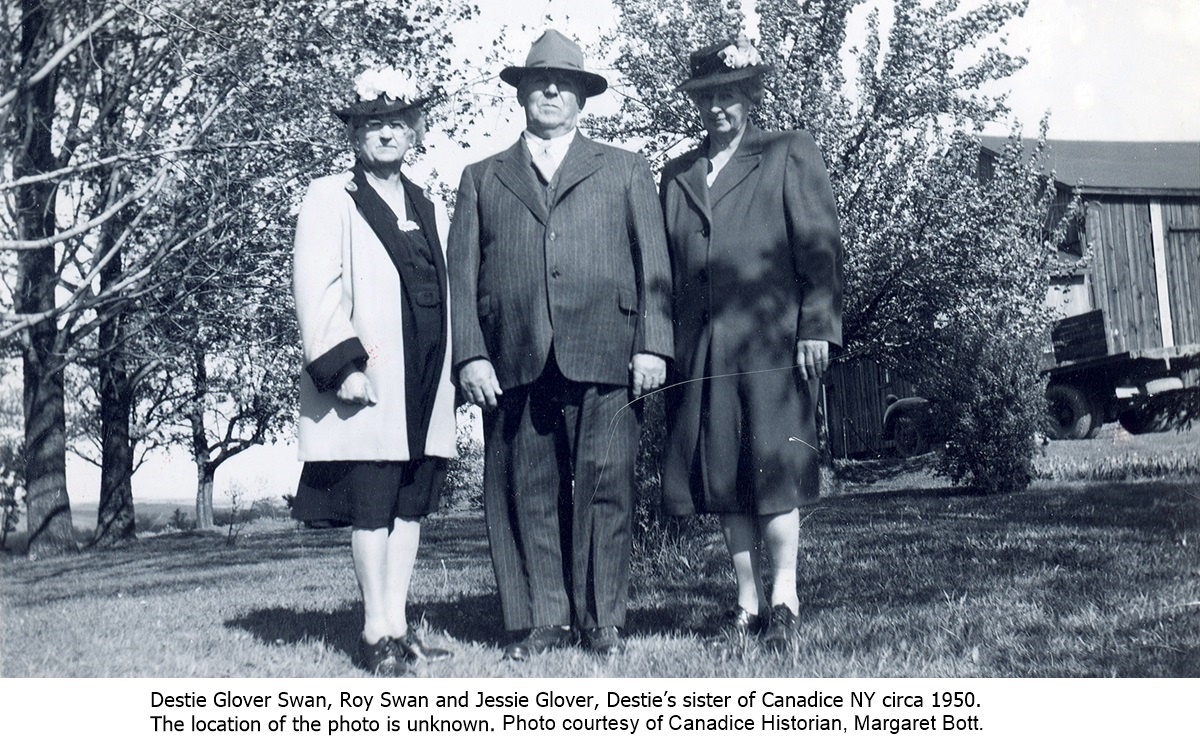This wide, rectangular black and white photograph features three older individuals posing in a grassy area with several tall trees in the background, some with flowers blooming. They are standing in front of a farmhouse and an old truck. The group consists of a man in the middle and two women on either side. The man, dressed in a dark pinstripe suit and a 1950s-style hat, also wears leather shoes. The women are adorned in thigh- and knee-length coats of different shades, and both wear floral hats. No one in the photo is smiling. The caption at the bottom, displayed over a white rectangle in black text, reads: "Dusty Glover Swan, Roy Swan, and Jesse Glover, Dusty's sister of Kennedy's, New York, circa 1950. The location of the photo is unknown. Photo courtesy of Candace historian Margaret Bott."